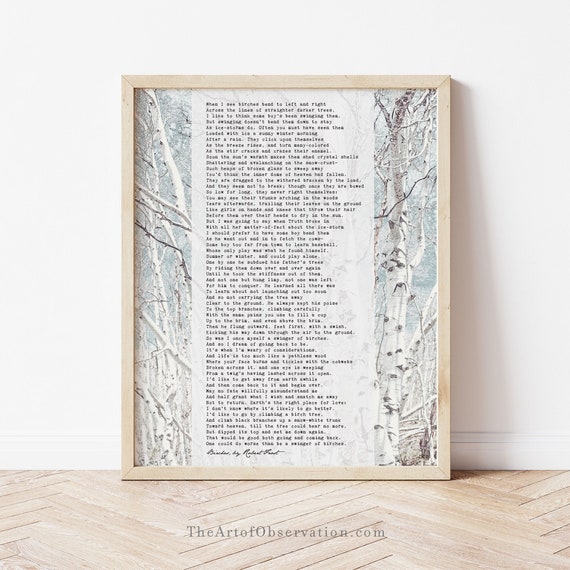The image showcases a piece of art that appears to be an advertisement for the website theartofobservation.com. The artwork is framed in a thin, light wood frame and is resting against a white wall on a hardwood floor with a diagonal pattern. The print features a serene, snowy landscape with tall, bare trees that have whitish trunks and numerous limbs, devoid of any leaves. Superimposed in the center of the scene is a transparent white rectangle filled with a poem or story written in small black lettering. The exact contents of the text are difficult to discern from the image, and the poem is signed in cursive at the end. The overall composition of the image suggests a wintery, contemplative theme, perfectly suited for promoting artistic and literary expressions.